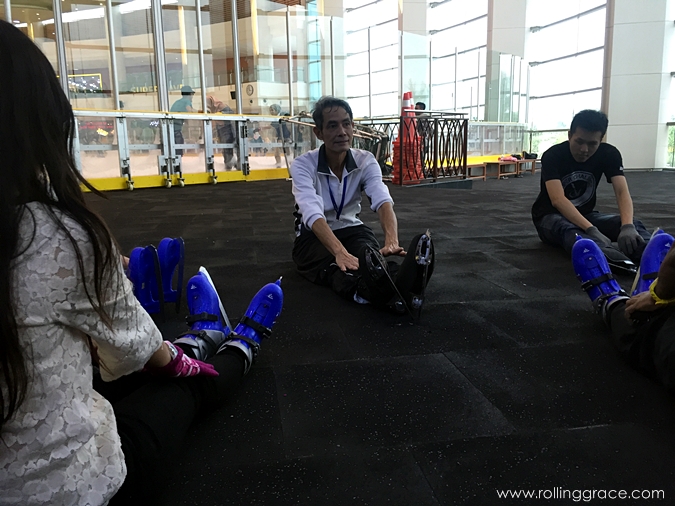The photograph depicts three individuals preparing to put on ice skates while seated on a black padded mat in what appears to be a gym or workout room. Two men, likely Asian, can be seen from the front while the back of a woman with long, straight black hair is visible on the left edge of the image. The individuals are equipped with blue and black ice skates, readily identifiable by the blades underneath. The man in the center wears a press pass ribbon around his neck. In the background, a curved glass wall separates the room from what seems to be an ice rink, and beyond this, more exercise equipment is visible. Additionally, the right side features a wall with columns and windows, allowing sunlight to stream into the room. A small black fence is present behind the central man, adding to the intricate details of the setting. The bottom right of the image displays the website www.rollinggrace.com.